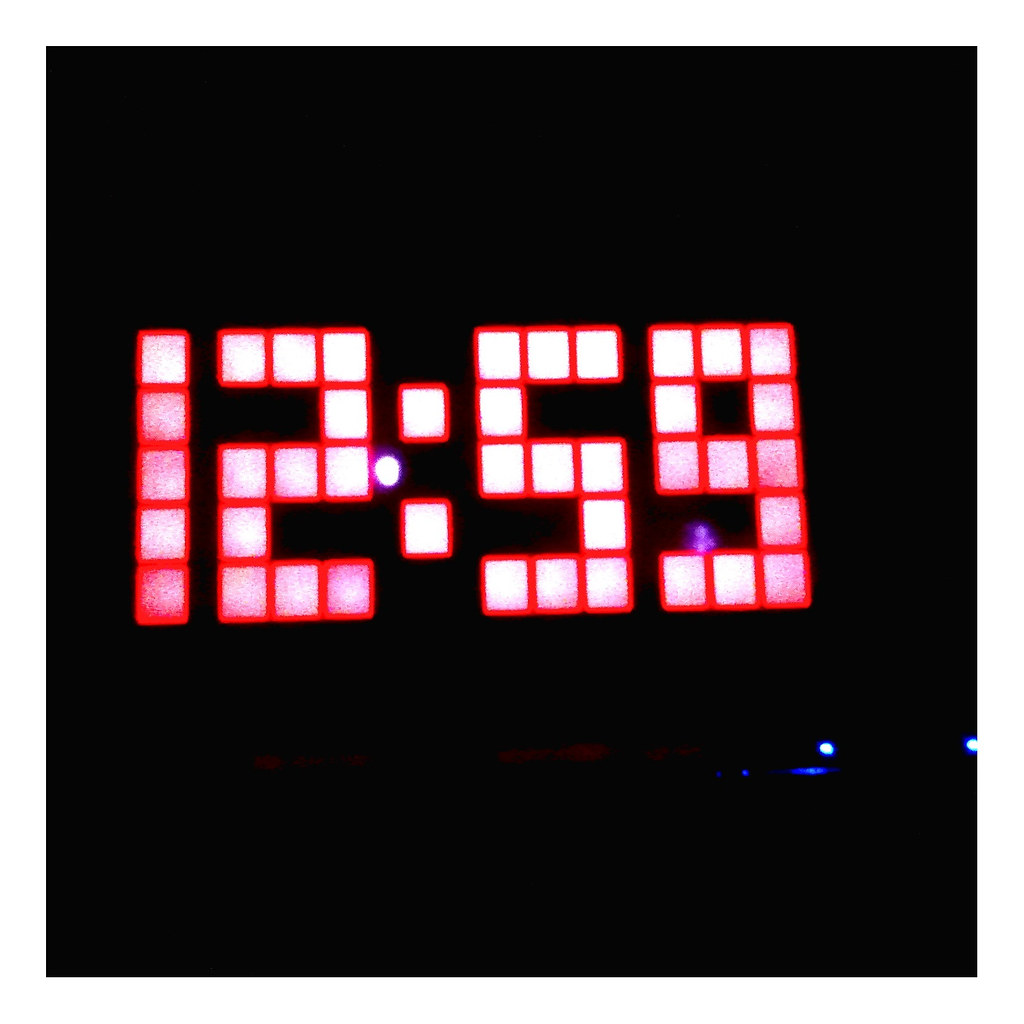The image is a realistic, square-shaped photograph, potentially taken at night or in a very dark place. The background is entirely black, resembling either a dark room or an outdoor setting at night. In the center of the image, digital clock-like numbers read "12:59," created from white squares with red outlines arranged in a grid pattern, three boxes wide by six boxes tall. These numbers stand out vividly against the dark backdrop. Additionally, there are a few small blue lights visible near the bottom right of the image, likely resembling flashlights or some subtle lighting source. The overall scene has no discernible people or other objects, adding to the mystery of its setting, which could be an arena, a digitally created environment, or another dark venue.